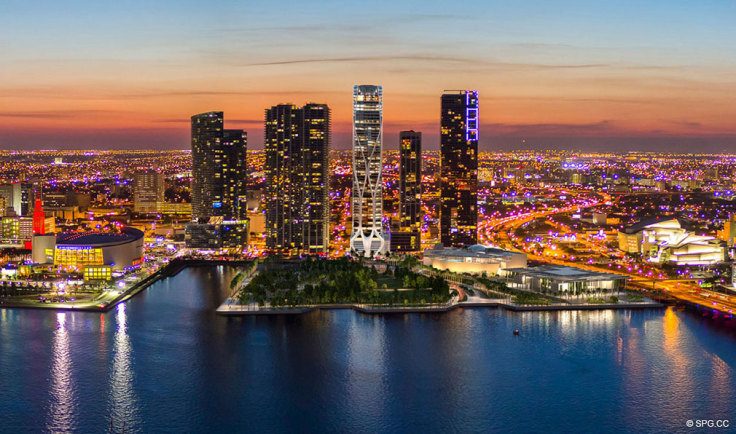This aerial photograph captures a sprawling cityscape just before sunrise or shortly after sunset, utilizing both natural and artificial light to create a vivid, full-color scene. The horizontally rectangular image showcases a mixture of black and white skyscrapers, predominantly concentrated in the center, each adorned with striking lights in hues of yellow, white, blue, and occasionally purple, particularly noticeable on a circular building on the far right. The bottom section of the image reveals a significant body of water, reflecting the urban lights and featuring a small boat in the bottom right corner. Roads, some appearing orange, weave through the city, and a man-made park area with abundant trees provides a lush green contrast amidst the urban structures. The sky transitions from a bright blue at the top to deeper oranges and purples near the horizon, adding to the scene's visual drama. The lower right corner of the photo contains a small text marking, reading "copyright SPG.CC."